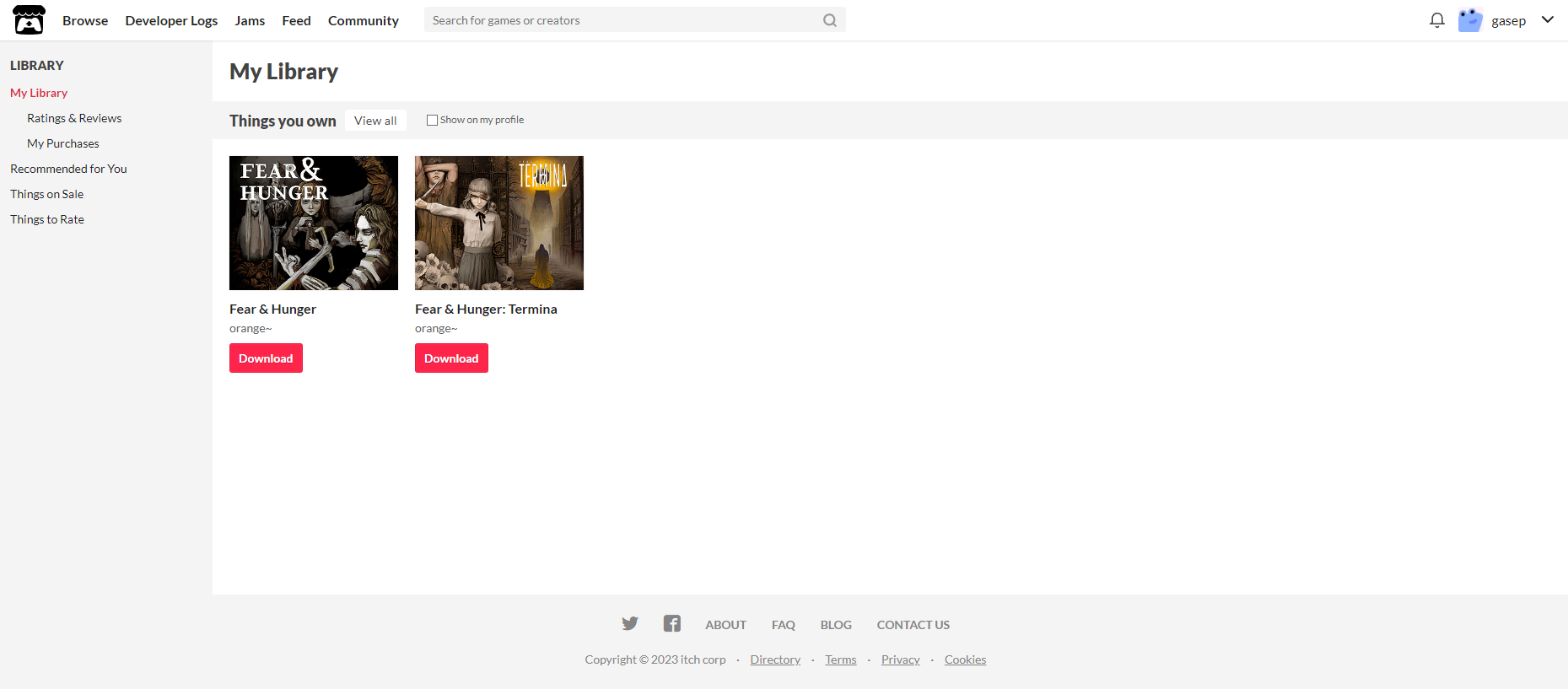A detailed caption for the described image could be:

---

The image captures a webpage from a game-centric site, prominently displaying a section titled "My Library". At the top of the page, a navigation menu includes icons and options such as a download icon, "Browse", "Developer Logs", "Jams", "Feed", "Community", and a search bar labeled "Search for games or creators" with a magnifying glass icon for search functionality. To the far right, the menu hosts a bell icon for notifications and a small user avatar accompanied by the username GASAP.

Beneath the main navigation, in bold print, is the title "Library". An underlined menu offers further options: "My Library", "Ratings and Reviews", "My Purchases", "Recommended for You", "Things on Sale", and "Things to Rate". Adjacent to this, a smaller, secondary menu repeats "My Library" with categories "Things You Own", "View All", and a checkbox option "Show on My Profile" for displaying items publicly.

The central portion of the webpage features two game titles. The first game, "Fear and Hunger," showcases an eerie, ghoulish artwork depicting a dark warrior with a sword and a witch-like woman. Below the image, the game title "Fear and Hunger" is accompanied by a download option. The second game, "Fear and Hunger Terminal," presents an aggressive-looking girl in warrior attire, extending her arms with rabbits on the ground behind her. Similarly, the game title "Fear and Hunger Terminal" appears below with a download option.

At the bottom center of the page, common site links and information are displayed, including social media icons for Twitter and Facebook, an "About" section, an FAQ, copyright information, and links relating to site policies such as directories and cookies.

---